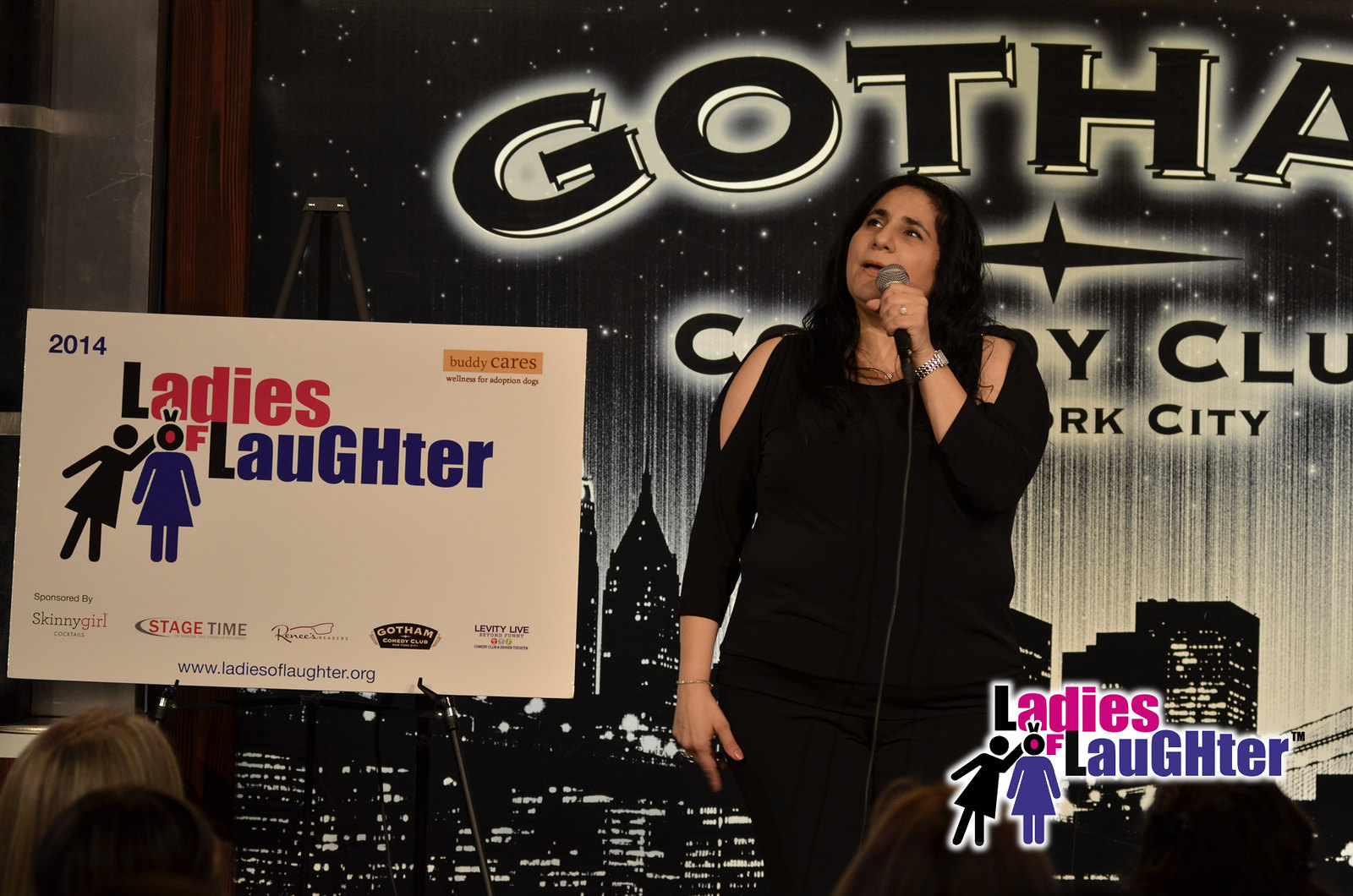A woman with long black hair is performing on stage, holding a microphone in her left hand and looking slightly upward. She is dressed in a black outfit that includes a three-quarter sleeve top with slit shoulders. The backdrop behind her is a black and white cityscape print labeled "Gotham Comedy Club, New York City." To her right, there is a stand holding a poster that reads "2014 Ladies of Laughter," featuring sponsor names such as Skinny Girl, Stage Time, and others. The poster also includes a website URL, www.ladiesoflaughter.org. In the lower right corner of the image, there's a logo with two female stick figures—one dark and one purple—with the text "Ladies of Laughter" in pink, purple, and black. Some audience members are visible at the bottom of the image, gazing at the performer.